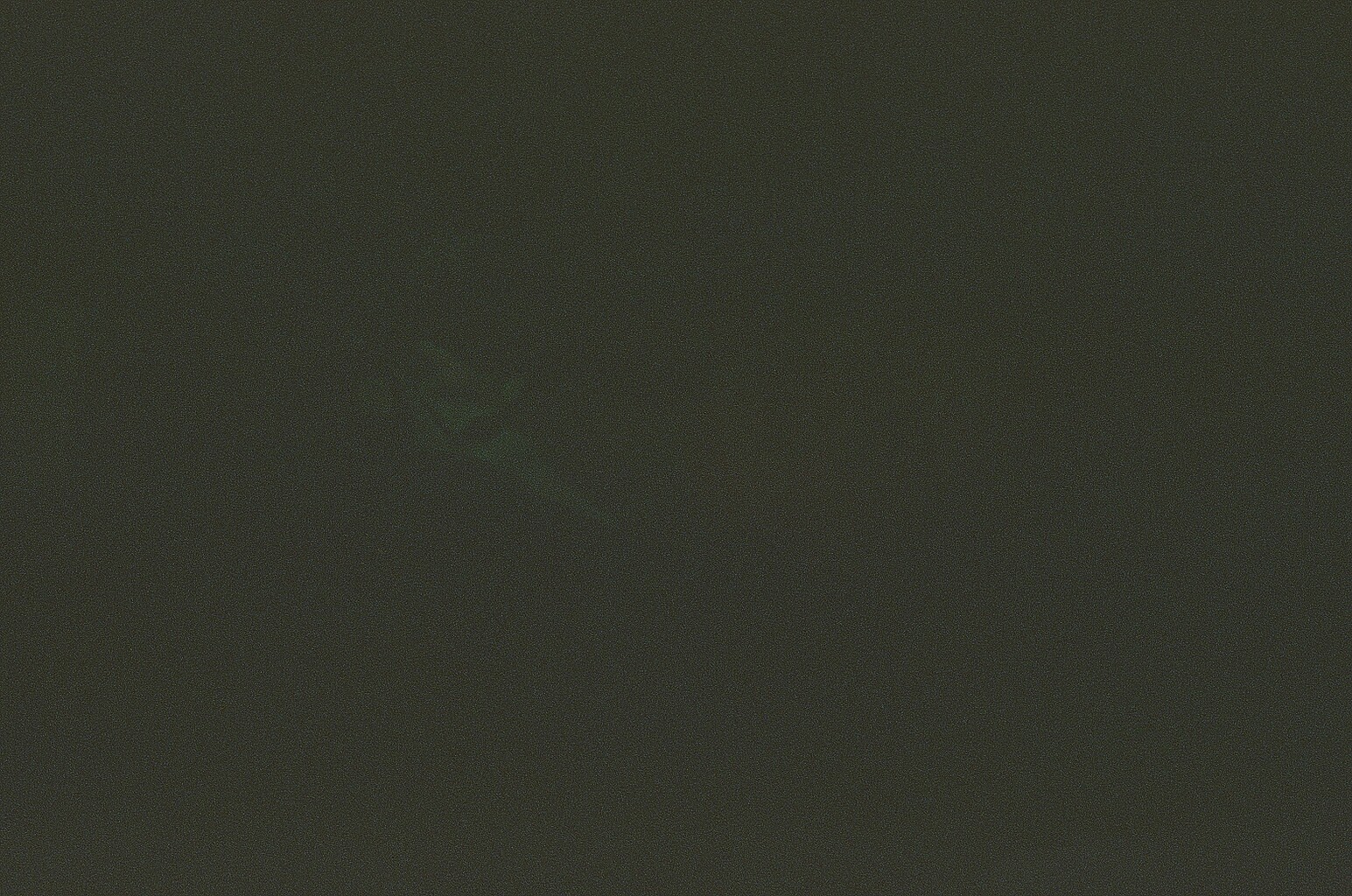The image exhibits an extremely dark, grainy background, primarily composed of deep green hues that gradually shift from darker shades at the top right to slightly lighter tones at the bottom left, creating a subtle diagonal gradient. Upon closer inspection, there is a faint triangular shape located slightly left of the center and midway up the vertical axis. This triangle, slightly lighter than its surrounding, has pointed angles and evokes the impression of a skull, particularly resembling a bird's skull, with possible dark spots that might be eye sockets. The texture of the image appears mottled, hinting at almost a carpet-like softness in the middle area, and includes sporadic dotted patterns. Despite the overwhelming darkness and the vagueness of the lighter area, the triangle stands out as the primary distinguishable feature amidst an otherwise indistinct, murky green backdrop.